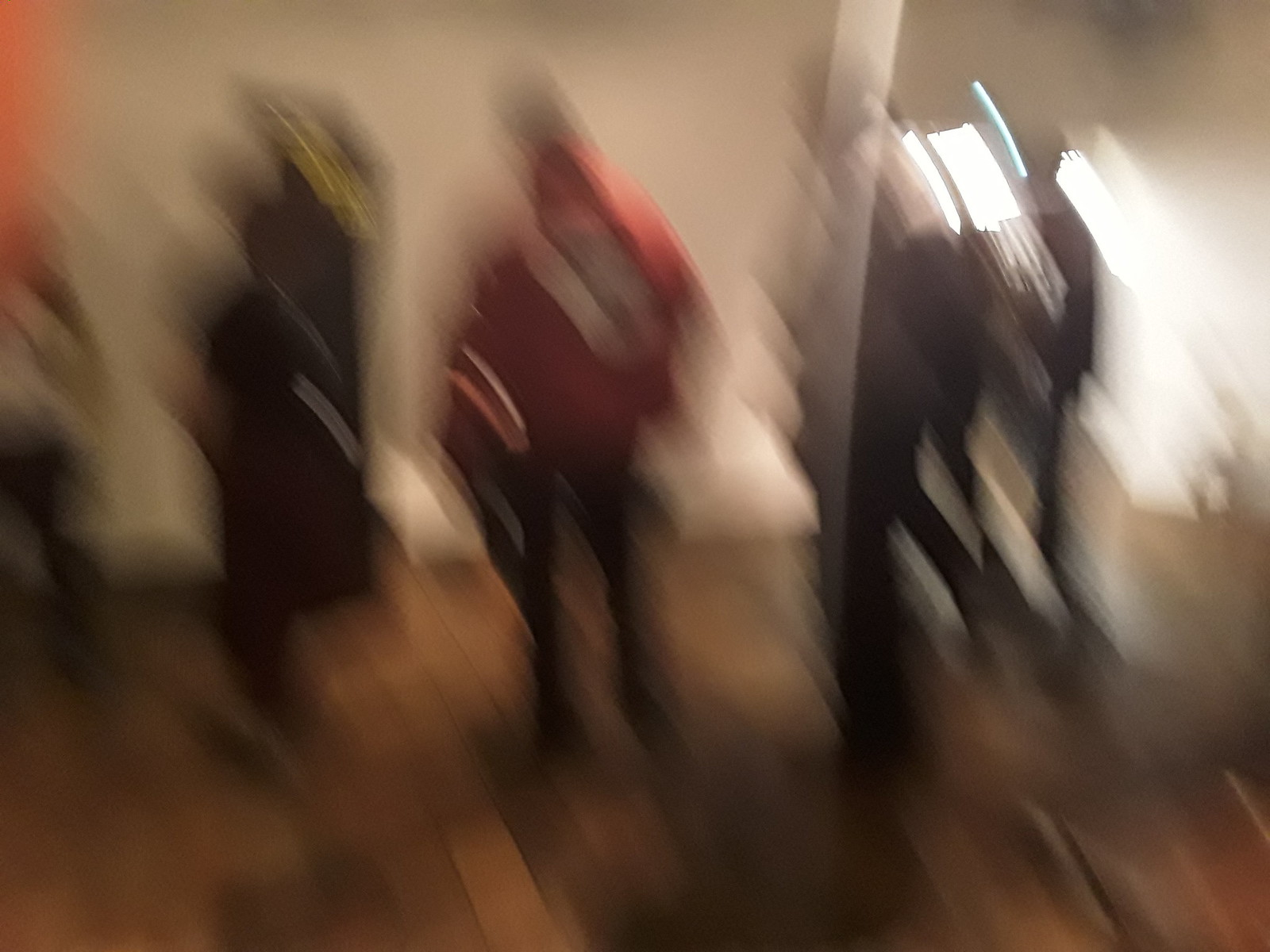This color photograph is notably blurred, making it challenging to discern specific details or elements within the scene. Despite the lack of clarity, it appears to depict an indoor setting with dark wood flooring. Various indistinct shapes suggest the presence of multiple people within the room. Central to the image is a figure seemingly clad in a red jacket. The walls of the room seem to be painted white. The photograph does not contain any animals, plants, flowers, trees, motorized vehicles, or mechanical objects, and there is no legible writing visible. Due to the significant blurriness, fine details and exact activities remain indeterminable.